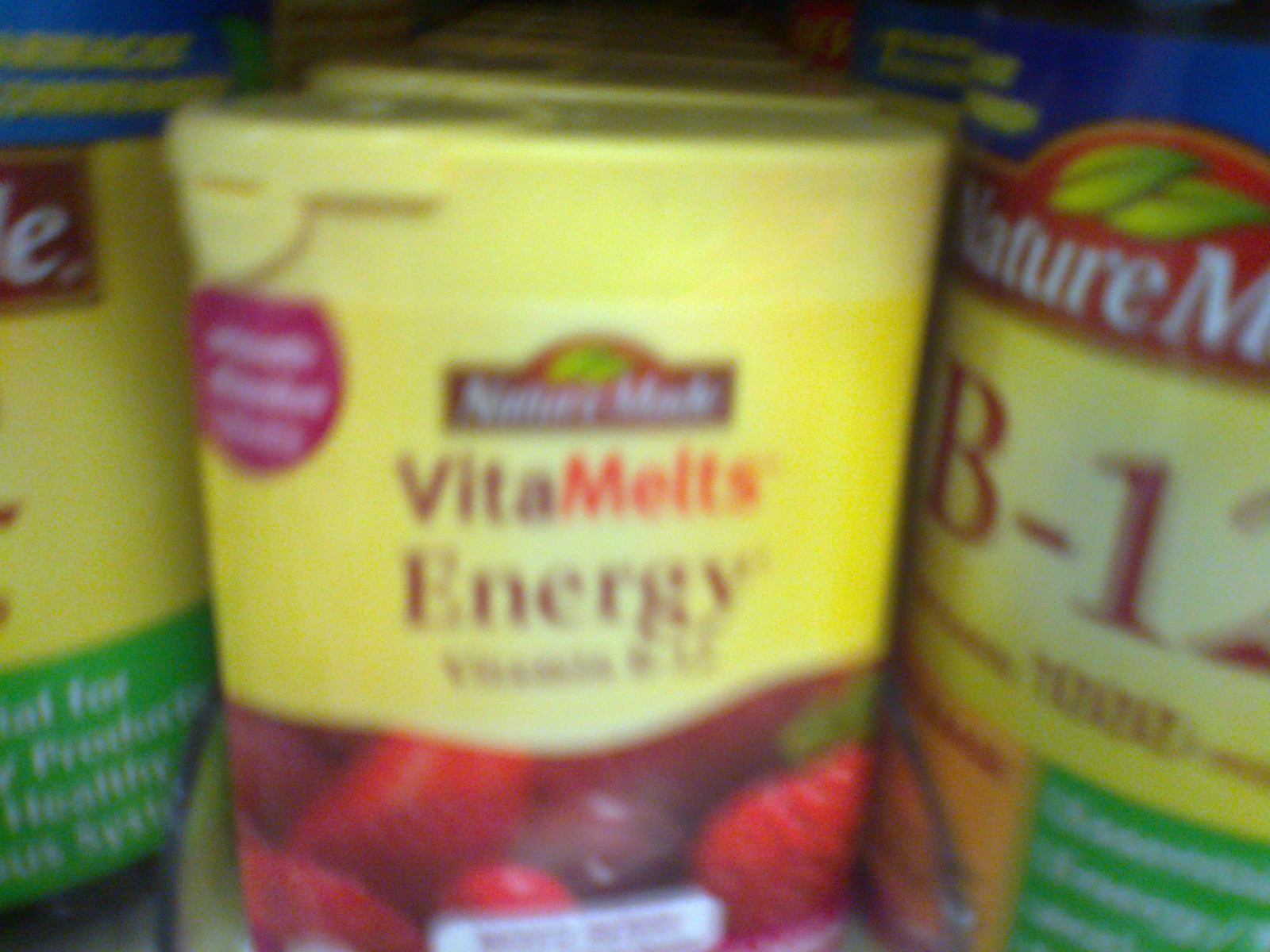This image depicts a blurry, indoor, color close-up photograph of vitamin packages on a display shelf, likely in a store. The image features three main packages, with the central one being the most identifiable. This middle package is a yellow, oval-shaped container with a prominent red round sticker at the top. The label reads "Nature Made" followed by "VitaMelts Energy." Below this text, the label includes images of strawberries, and possibly other fruits, indicating the flavor. On the left edge of the image, a partial view of another container is visible but not clear enough to discern details. On the right side, a blue-topped container can be seen with "Nature Made" written in white, and below that, in a yellow section, it says "B12." Both the left and right rows of products extend into the background, confirming the shelving setup typical of a store display.